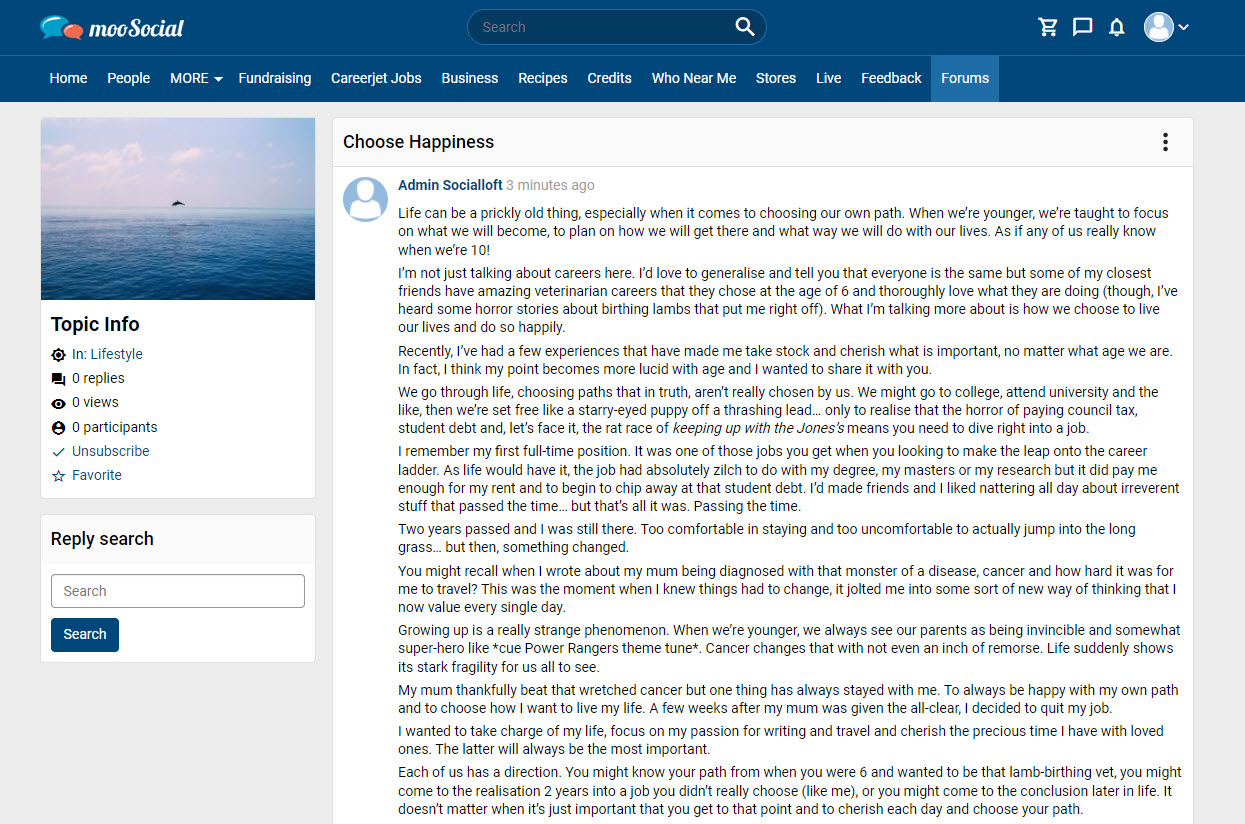This is an image from a website called Move Social, featuring a post by the admin titled "Choose Happiness," published three minutes ago. The post eloquently discusses the challenges of navigating life and making choices that lead to personal fulfillment. It reflects on how, from a young age, we are often directed to focus on future goals and careers, sometimes as early as age ten, despite the complexities and uncertainties of life. The author shares anecdotes about friends with successful careers in veterinary medicine, chosen with conviction at a very young age, while also acknowledging the distressing experiences that can come with such paths. The core message stresses the importance of cherishing what truly matters and striving for happiness, regardless of age or the predetermined paths we follow. The image likely complements this thought-provoking and insightful narrative on the pursuit of a life well-lived.